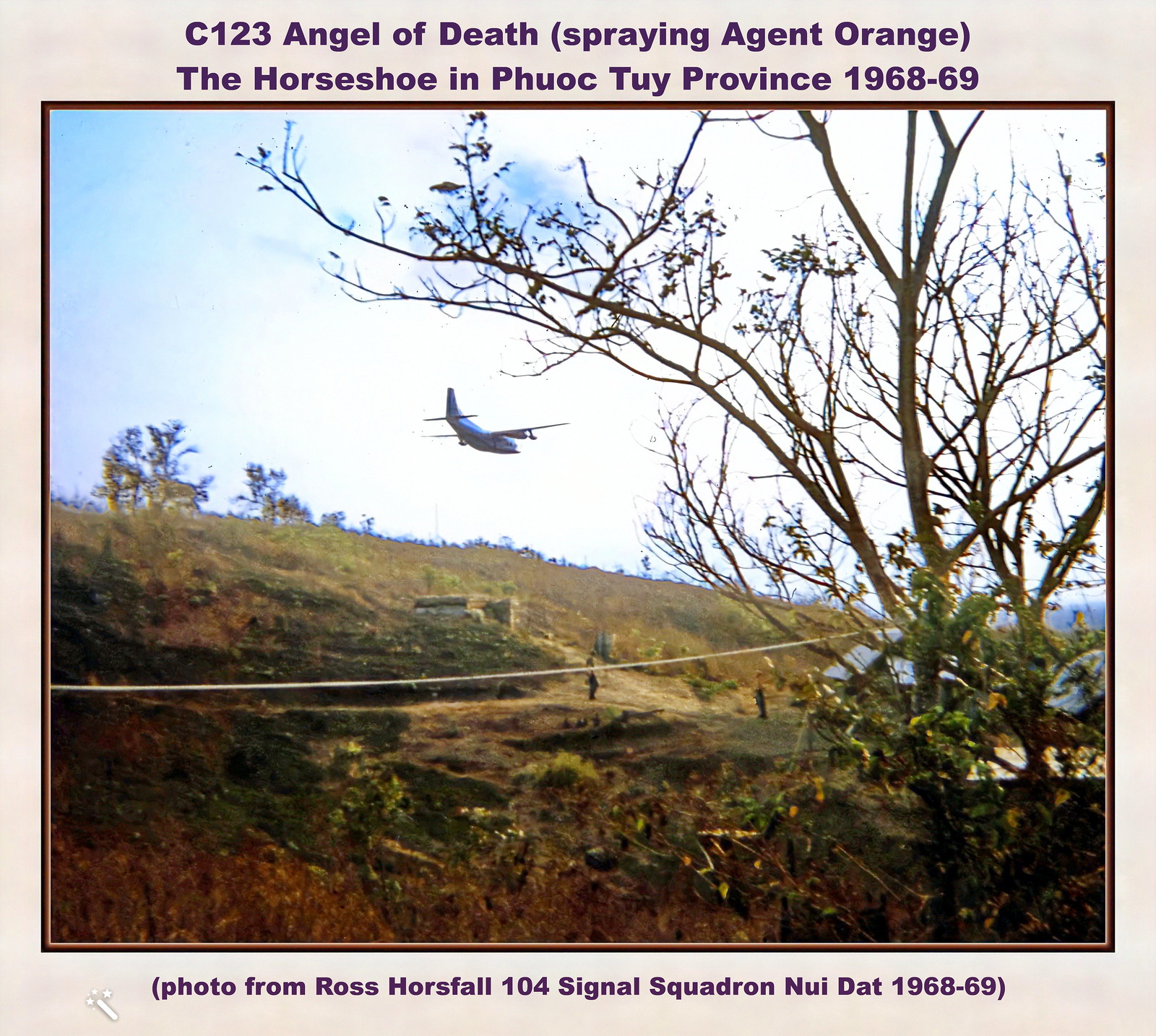The image is from the Vietnam War and depicts an outdoor area with a significant historical context. Dominating the scene on the right is a large tree, while the middle left features an open plain that transitions into a hillside adorned with more trees under a blue sky. A distinct white line runs diagonally from the bottom left to the right side of the image, possibly denoting a pathway or the area being targeted. The landscape displays varied green and yellow hues, suggesting a mix of grass and other vegetation, and hinting at a springtime setting.

An airplane, identified as the C-123 "Angel of Death," is depicted spraying Agent Orange over the area, with context provided by the purple text at the top of the photograph that reads: "C-123 Angel of Death spraying Agent Orange. The Horseshoe in Phuoc Thuy Province 1968 to 69." Additional text at the bottom notes: "(photo from Ross Horseville, 104 Signal Squadron, Nui Dat, 1968 to 1969)."

The photograph is framed by a cream-colored border followed by a brown one, giving it a vintage or archival appearance, possibly originating from a book or a collection.